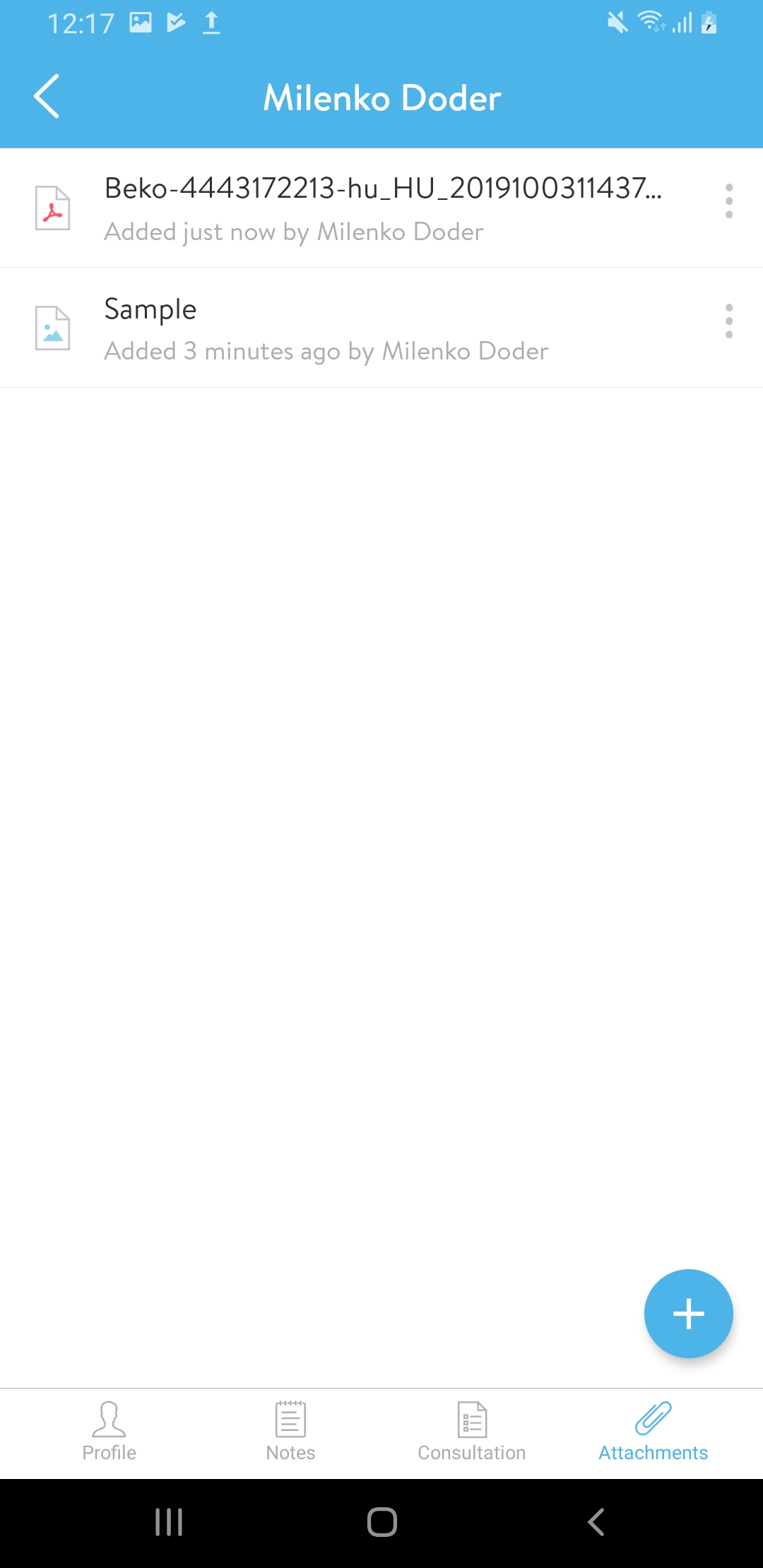A screenshot from an Android phone displays a screen from an unspecified app. At the top, the name "Milenko Doder" is prominently featured, indicating ownership or authorship. The background of this top bar is blue, offering a contrast to the otherwise white page. Below the name, two files are listed: one is a PDF and the other appears to be an HTML file. Both files are marked as "added just now" by Milenko Doder. Each file entry includes an ellipsis button for more options. At the bottom of the screen, a navigation bar showcases tabs labeled "Attachments," "Consultation," "Notes," and "Profile," with the "Attachments" tab currently open. A prominent plus button in the bottom right corner suggests the ability to add more files or content. The overall layout and design elements hint at a professional or organizational tool, potentially for managing client or patient information, as suggested by the presence of a "Consultation" tab.